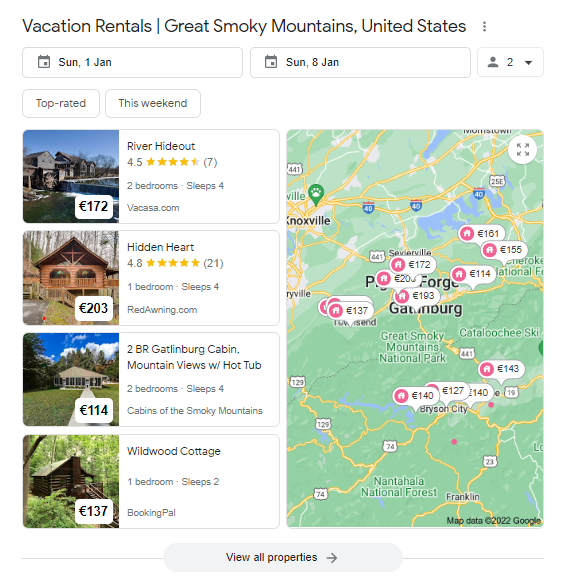**Detailed Caption:**

The image depicts a vacation rental application interface focused on listings in the Great Smoky Mountains, United States. The screen displays the trip details, showing a stay from Sunday, January 1st to Sunday, January 8th, with small calendar icons to the left of each date. The journey is planned for two travelers, as indicated by the person icon with the number '2'. Additionally, there are filter buttons labeled "Top Rated" and "This Weekend."

On the right side of the screen, there is a map highlighting a rural area with winding yellow roads and a few lakes. Key locations such as Knoxville, Tennessee, and other nearby towns are marked. The property prices are shown in euros, and various lodging options are marked with pink circles that contain white house icons.

To the left of the map, four vacation rental results are visible, each accompanied by a photo:
1. **River Hideout** - A lodge with 4.5 stars, offering two bedrooms and accommodating up to four people. It is listed on Vacasa.com for 172 euros, with seven reviews.
2. **Hidden Heart** - A covered bridge-style property with a rating of 4.8 stars based on 21 reviews, featuring one bedroom and sleeping up to four people. It is available on Redawning.com for 203 euros.
3. **Gatlinburg Cabin, Mountain View with Hot Tub** - This two-bedroom cabin sleeps four and is available through "Cabins in the Smoky Mountains" for 114 euros.
4. **Wildwood Cottage** - A cozy log cabin with one bedroom, suitable for two travelers. It is listed on Booking Pal.

Below these listings is a button labeled "View All Properties" with an arrow pointing to the right, suggesting there are more rental options available beyond the initial four displayed.